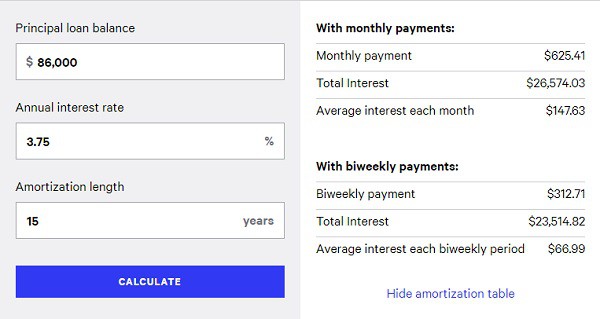The image depicts a loan calculator interface. On the left side, there are three rectangular input fields. The first field, labeled "Principal Loan Balance," has an entered value of $86,000. The second field, labeled "Annual Interest Rate," shows an input of 3.75%. The third field, labeled "Amortization Length," displays a period of 15 years. Below these input fields is a blue "Calculate" button with white text.

On the right side, the calculation results are prominently displayed. In large, bold letters, it indicates the monthly payment details: a monthly payment of $625.41, total interest of $26,574.03, and an average monthly interest of $147.63. Additionally, it provides information for a bi-weekly payment plan: a bi-weekly payment amount of $312.71, total interest of $23,514.82, and an average bi-weekly interest of $66.99. At the bottom right corner, there is a section labeled "Amortization Table" in blue text.